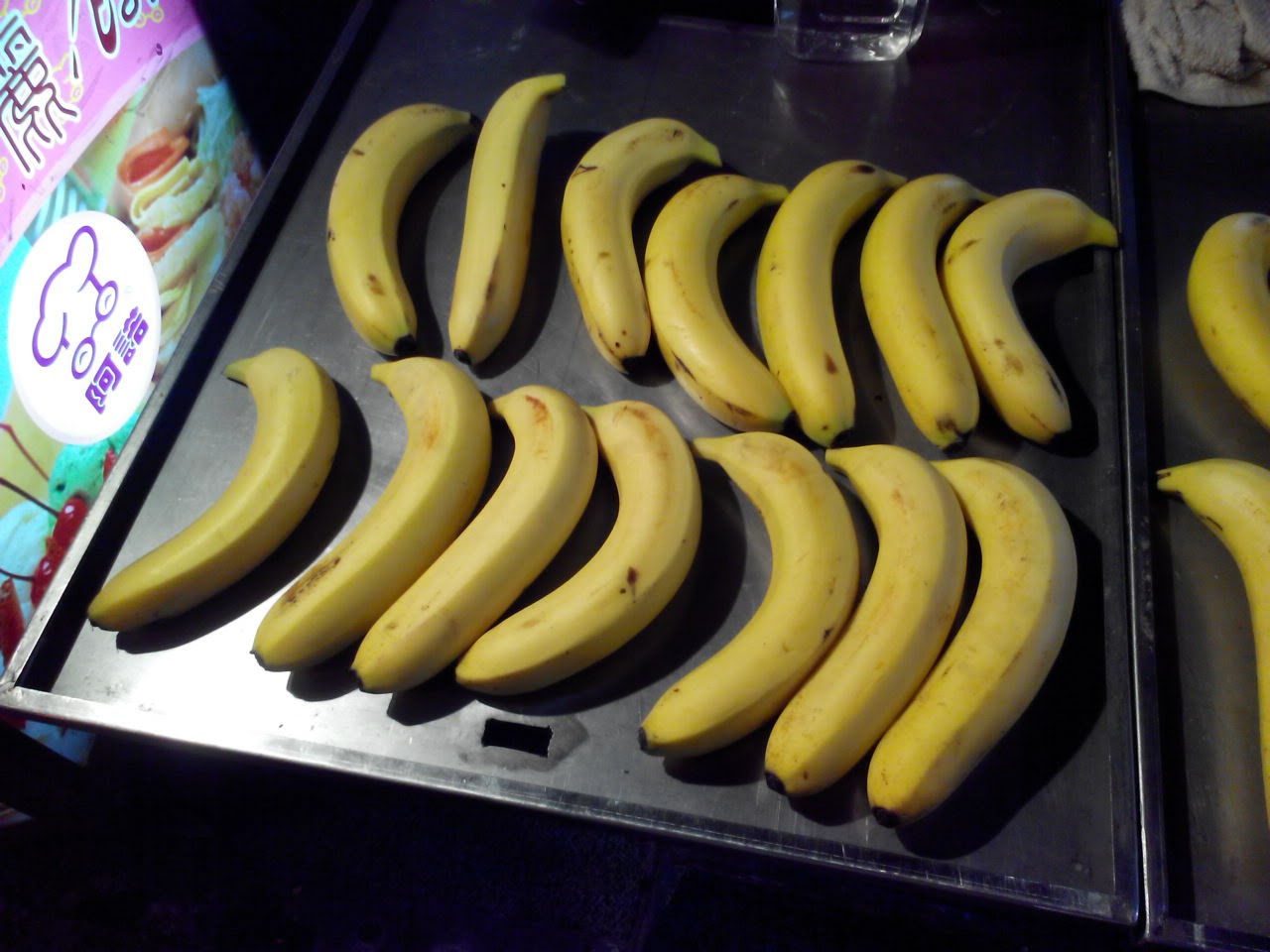The image depicts a digital photograph taken indoors, showcasing a black table prominently in the center. The table is adorned with a neat arrangement of bananas: two parallel rows with the upper row consisting of eight yellow, fairly ripe bananas with dark spots, and the lower row comprising seven bananas, their tops oriented in opposite directions. To the right side of this table, a second table can be seen, holding two additional bananas, one positioned above the other. On the upper left corner is a distinct illuminated banner featuring dark blue Asian script and a circular icon with a chef's hat and glasses, alongside more blue script. The banner also displays a brownish tan food item, whose specific nature is unclear. The black table also supports a square glass container towards its back, visible yet slightly off-center in the photograph.